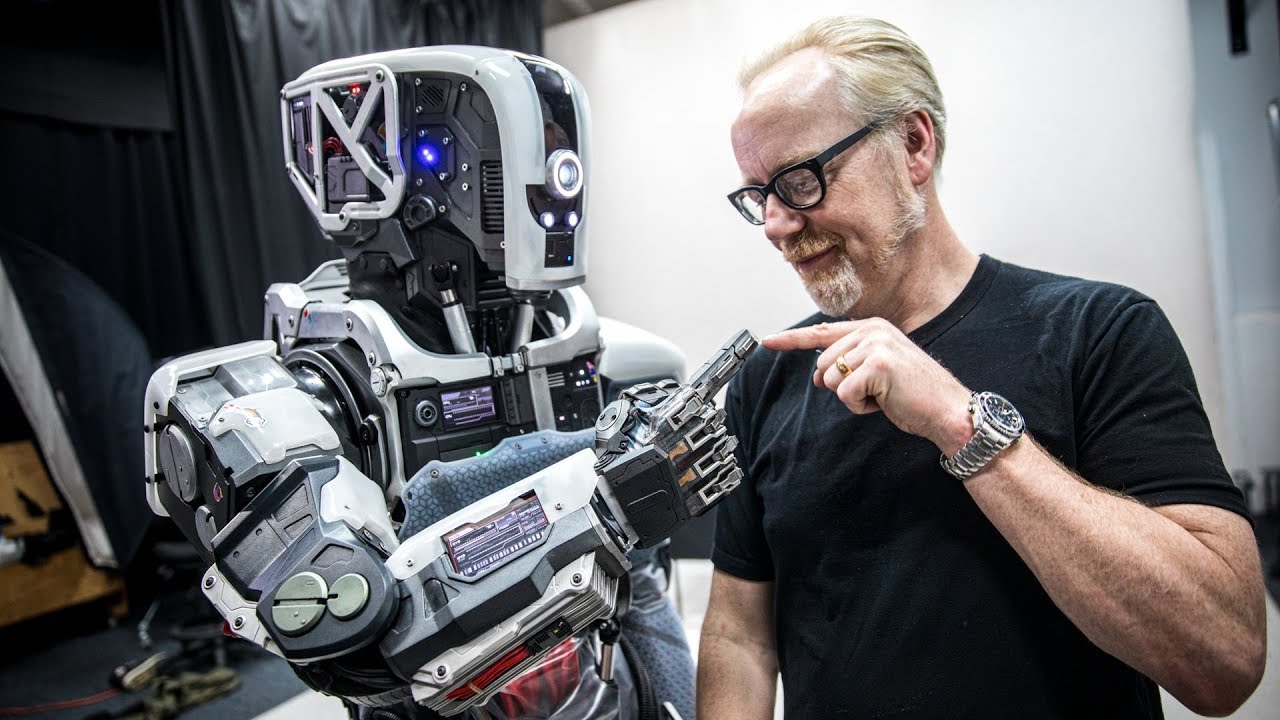This photograph captures a poignant interaction between a middle-aged man and a sophisticated humanoid robot. The man, positioned on the right, appears to be Caucasian in his late 50s or early 60s. He sports a black short-sleeved t-shirt, black rimmed glasses, a silver watch on his wrist, and a gold wedding band. His receding blondish hair transitions into a white beard and goatee, lightly tinged with reddish hues and revealing his freckled complexion. The man gently smiles as he gazes down, extending his left hand to touch fingertips with the robot.

The robot on the left side of the image, exhibits a high-tech, humanoid design with two arms and a distinct lack of human facial features. Its head, a curved oblong shape, features a prominent circular light in the center of its flat front. The robot’s predominantly gray and black body is adorned with various controls, blue and red lights, and hydraulic mechanisms around its neck. Notably, red wiring is visible near its midsection. The robot’s right hand, detailed with articulated fingers, mirrors the man's gesture by extending its mechanical finger to meet the man's touch.

The backdrop of the image presents a stark, contrasting studio environment with a white drop background flanked by a black curtain and some indistinct objects in the left corner. This visually emphasizes the intimate connection between human and machine, highlighting advancements in robotic technology and the human fascination with it.